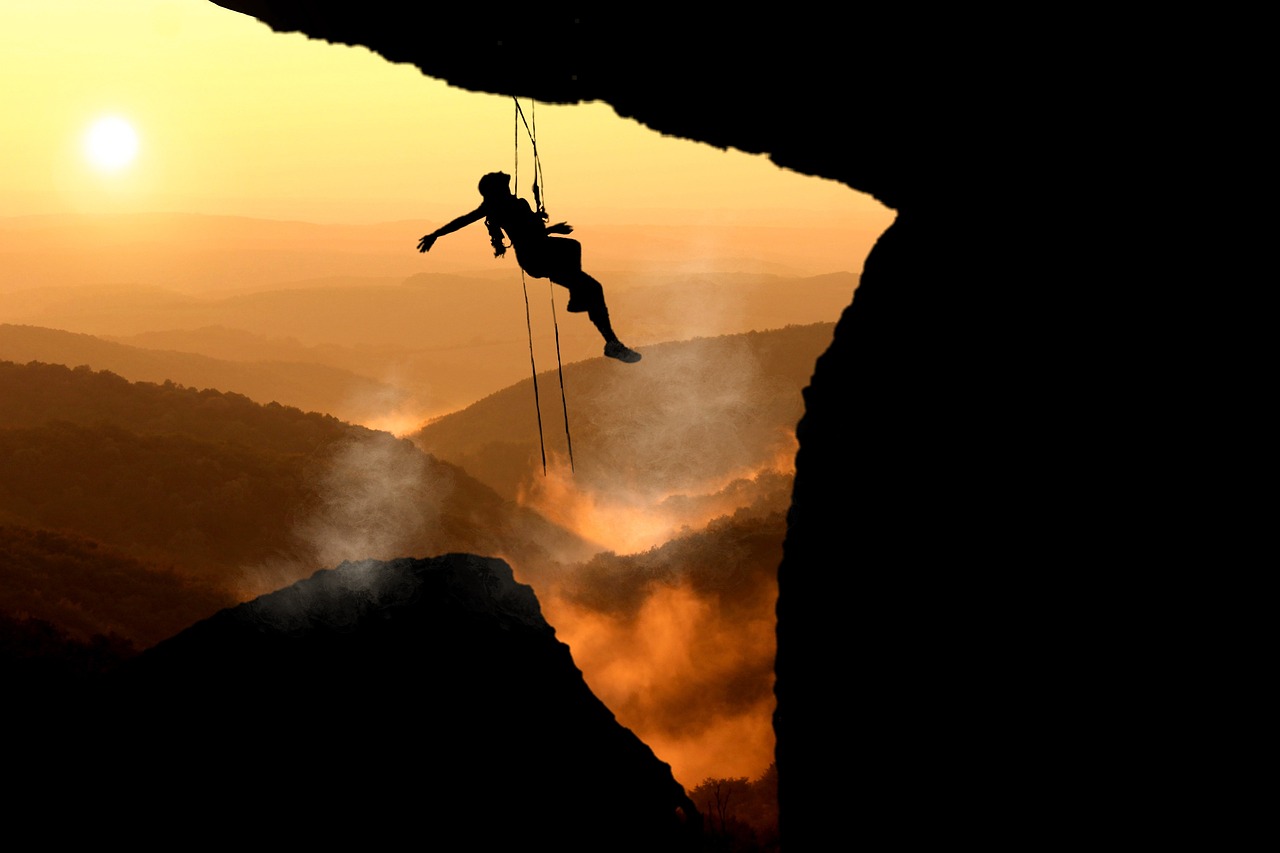Set against a spectacular outdoor backdrop, this high-contrast photograph captures a climber silhouetted against the sun, which sits bright in the upper left corner. The climber, who appears to be female, hangs precariously by security ropes from a craggy rock outcrop that juts outwards. Her silhouette is rendered in black due to the intense backlighting from the sun, which casts a stunning golden glow across the scene. This bright, yellow-orange sky creates a dreamlike atmosphere, blending with the silhouetted mountainous landscape that stretches into the distance. The rock formation surrounding her, both above and beneath, is rugged and forms a dramatic natural frame around her. In the background, a series of misty hills and dense forests soften the ruggedness of the cliff, completing this mesmerizing snapshot of human endeavor against nature's majesty.